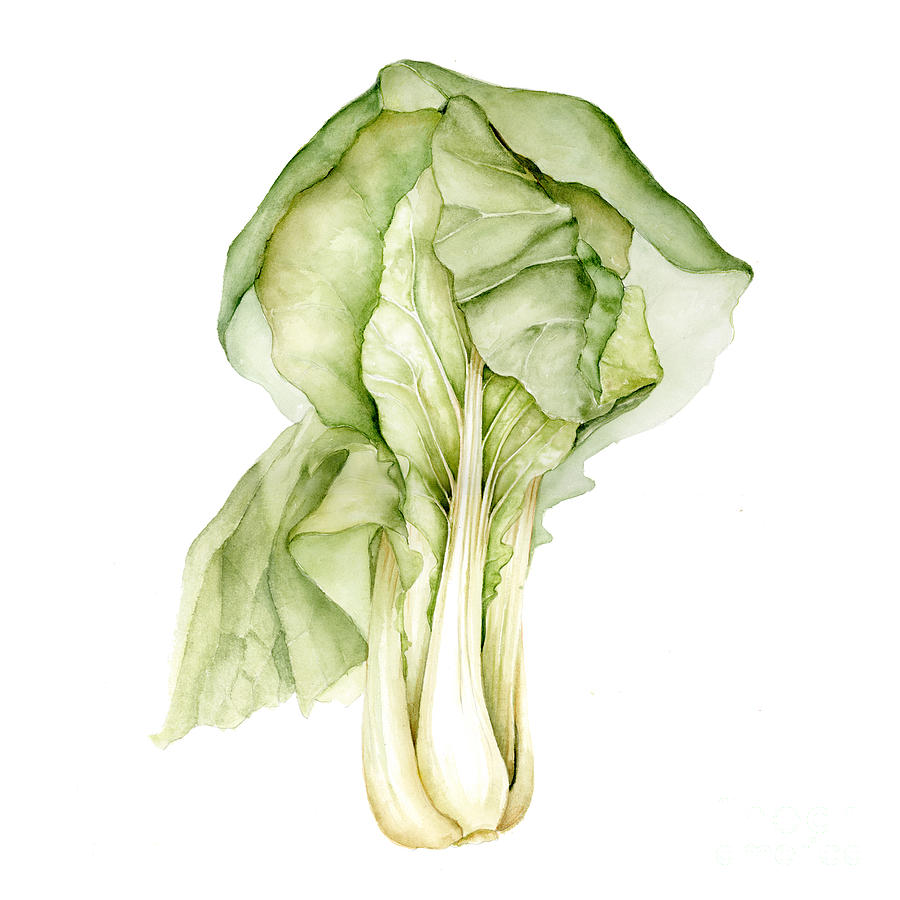The image depicts a watercolor painting of a bok choy vegetable against a white, rectangular background. The painting is characterized by its soft, fluid brush strokes that give a delicate, airy feel to the composition. The bok choy’s base comprises thick, interconnected white bulbs or stems, resembling vertical cylinders that merge together. From this base, the plant extends upward into luscious, expansive green leaves that exhibit various shades of green and hints of beige. Prominent veins are visible in the leaves, adding texture and detail. The main leaf at the top has a somewhat mushroom shape, while a smaller, tubular leaf appears to be folded down on the bottom left, paler in color. Overall, the painting captures the leafy, layered structure of the bok choy, presenting it with both accuracy and artistic grace.